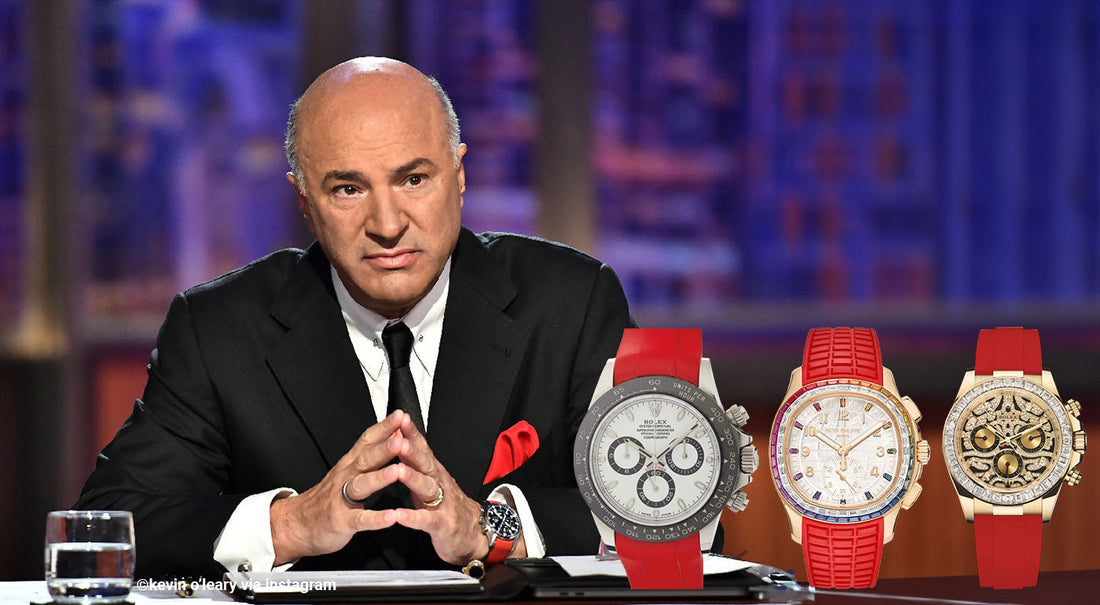This is a detailed photograph of Kevin O'Leary, one of the judges from Shark Tank, captured in a seated position and attentively observing a pitch. Kevin O'Leary is identifiable by his name watermarked with a copyright symbol in the lower left corner. He is dressed in a classic black tuxedo with a white collared shirt, a black bow tie, and a red pocket square. His attire is complemented by two rings, one on each ring finger, and a distinctive red wristwatch. To his left, there is a glass of water. The background is a blue-purple hue, suggesting a possible city setting, indicative of a formal or talk show environment. Overlaying the photo are three prominent watch models, all featuring red straps and closed bands. One watch resembles a tire track on the wristband, another has three different time zones with a gray rim, and the third showcases intricate gear designs with black and gold accents. The image also contains writing that reads "Kevin O'Leary via Instagram" in small white letters.